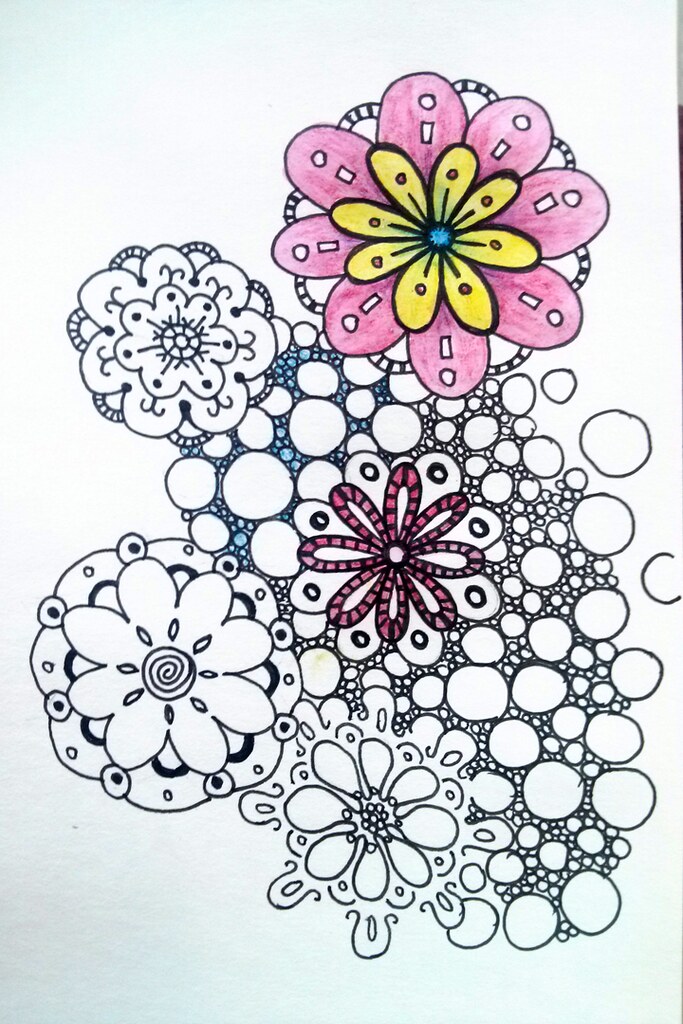The image bears a striking resemblance to a meticulously detailed page from an adult coloring book or a digitally created composition that might evoke memories of designs made with a Spirograph. Rendered in precise black ink on white paper, the artwork showcases an intricate array of geometric shapes, primarily circles, forming flower-like patterns. While the majority of the piece remains monochromatic, a portion has been vividly colored. One prominent flower features an outer ring of pink petals with a subsequent ring of yellow petals adorned with darker pink dots and a blue center. Another notable flower presents a center that resembles a tied bow, with the bow portion colored in light red. Scattered throughout the image are clusters of small circles perhaps resembling bubbles, some of which are colored in blue, particularly in the top-left area. The collective depiction offers a mesmerizing blend of geometric precision and bursts of color, expertly balancing structure and creativity.